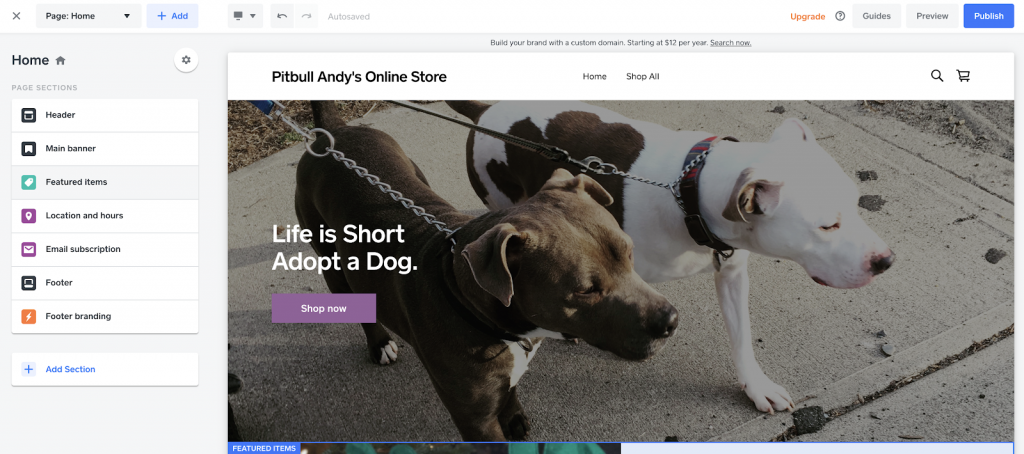In this image, we see a website interface designed for creating or editing a webpage. 

At the top right corner, there's a blue button labeled "Publish" in white text. Next to it, moving left, are the options "Preview," "Guides," and an orange "Upgrade" button. On the top left, there is an "X" symbol, followed by "Page Home" and an option to "Add" which has a plus symbol next to it. The background color of this header section is blue.

The central portion of the image features a photograph of two dogs being walked by their owner. The dog on the right is mostly white with some brown spots on its right side. It has a black nose and ears that are a mix of brown and white. This dog wears a collar that is a black and red combination. The dog on the left is predominantly brown but has white fur on its chest and feet.

In front of the photo, there is text that reads "Life is short, adopt a dog." Beneath this text, a purple rectangular box with white text says "Shop Now."

On the far left side of the image, a vertical menu lists various page categories: "Header," "Main Banner," "Featured Items," "Location and Hours," "Email Subscription," "Footer," "Footer Branding," and at the very bottom, "Add Section."